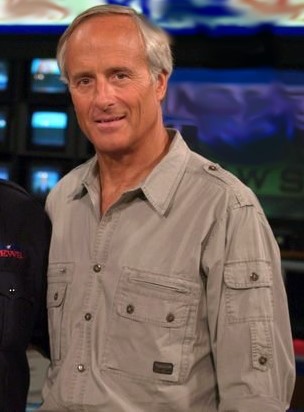In this close-up photograph, animal expert Jack Hanna, recognizable by his short, thinning gray hair parted to the side, stands with a gentle smile. He is wearing a tan, long-sleeved, cargo-style button-up shirt adorned with multiple pockets, including two on the chest and one on the left arm, and is paired with copper buttons and shoulder straps that also have buttons. Jack has his arm around another person, who is somewhat obscured but appears to be dressed in a black suit jacket. In the background, there are multiple monitors displaying various colors, suggesting that they are in a news station studio. The backdrop includes a hint of a blue area to the right, contributing to the high-tech studio environment.